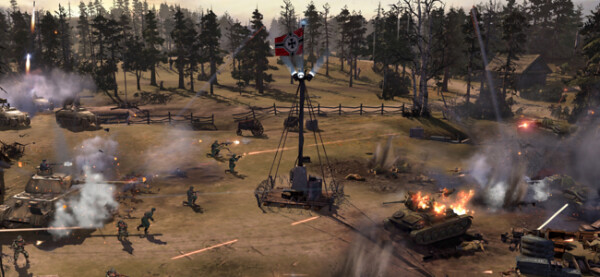This image depicts an intense scene from a video game, likely Battlefield or Call of Duty, featuring a battleground where multiple soldiers are engaged in capturing a flag. At the center of the expansive area stands a flagpole, currently displaying a flag that bears a striking resemblance to Nazi insignia: a red background with a white circle and a black cross in the middle, reminiscent of the Iron Cross. On one side, there are six soldiers actively firing their weapons, supported by an intact tank. The opposing side appears to be at a disadvantage, with their tank destroyed and fewer soldiers visible.